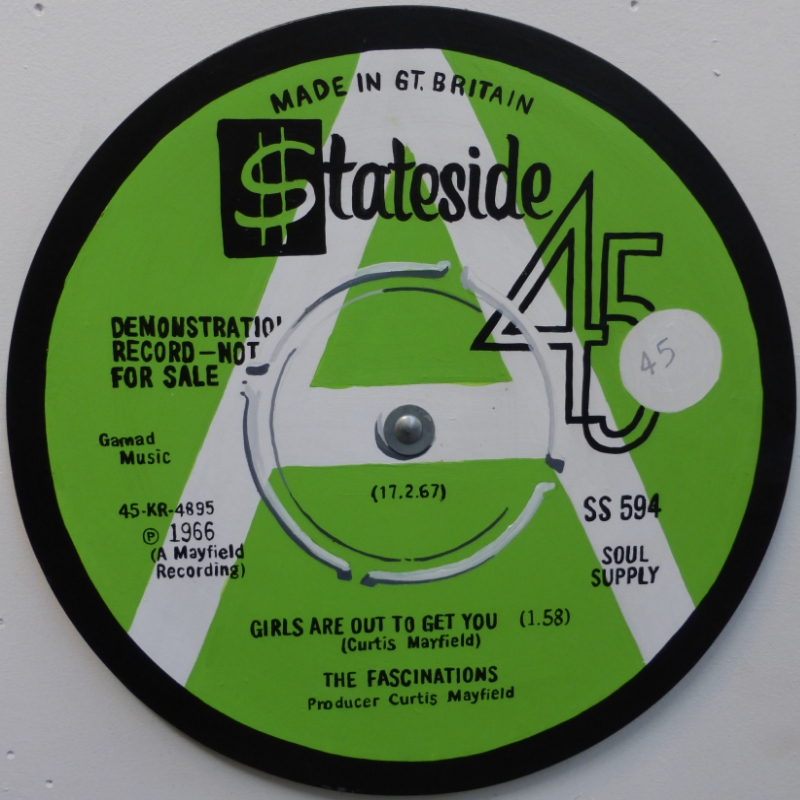This is a photograph of a demonstration record, not for sale, made in Great Britain. The record has a black border surrounding a light gray background, with a prominent lime green inner circle. Dominating the green section is a large uppercase letter "A" in white. At the top, the text reads "Made in Great Britain," followed by a logo for Stateside with the 'S' stylized as a dollar sign. A large "45" is visible on the right side of the circle. At the center, near the hole, there's a date: February 17, 1967, alongside a serial number 45KR4895 and a circled "P" marked 1966, indicating it as a Mayfield Recording. At the bottom of the record, the title "Girls Are Out to Get You" is listed, along with a running time of 1 minute and 58 seconds, credited to Curtis Mayfield and The Fascinations, with Curtis Mayfield noted as the producer.